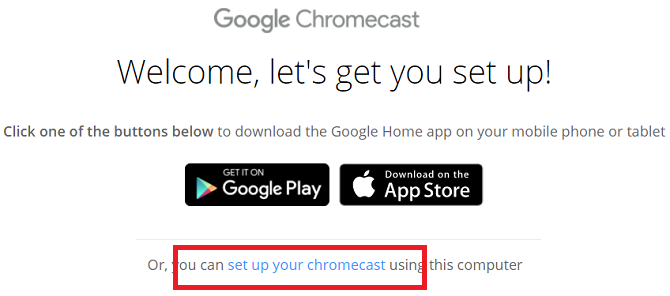This image is a screenshot of the initial setup page for Google Chromecast. The screen prominently displays a welcoming message: "Welcome! Let's get you set up." Below this message are instructions prompting the user to download the Google Home app on their mobile phone or tablet. Two buttons are visible beneath these instructions: the Google Play button on the left for Android users and the Apple App Store button on the right for iOS users. At the very bottom of the page, there's an additional option for setting up the Chromecast using a computer, accompanied by text that reads, "Or you can set up your Chromecast using this computer." Notably, there is a red outline bar that has been superimposed over this part of the text, which is not part of the original setup page and appears to have been added after the screenshot was taken. The image itself is relatively small, suggesting it might have been cropped and that more content is likely present on the full welcome page.